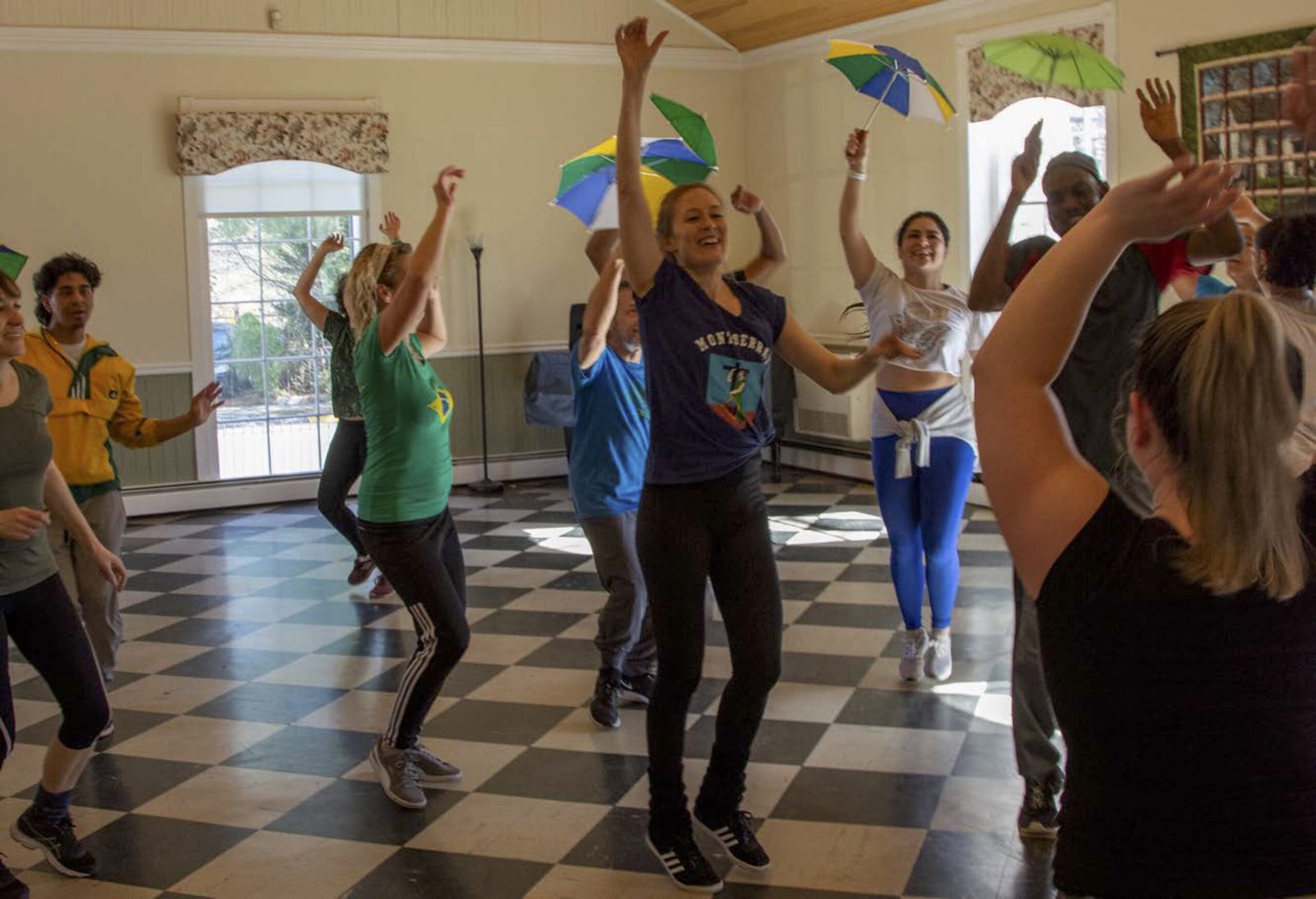The photograph captures a lively dance or exercise class in a spacious room with a checkerboard floor of light and dark brown tiles. The room features light brown walls with dark forest green wainscoting, and tapestry decorates one side, while two windows adorned with decorative curtains let in ample natural light. 

The class consists of 12 people, predominantly women, donned in typical exercise attire—leggings, T-shirts, and sneakers—while engaging in animated dance moves with arms and knees raised. Most are smiling and immersed in the routine, some holding small umbrellas in colors like blue, white, yellow, and green, adding a playful element to the scene. 

A lamp stands in the background, and at the front of the room, an instructor in a black shirt with a high ponytail demonstrates the moves, directing the group's energetic performance.